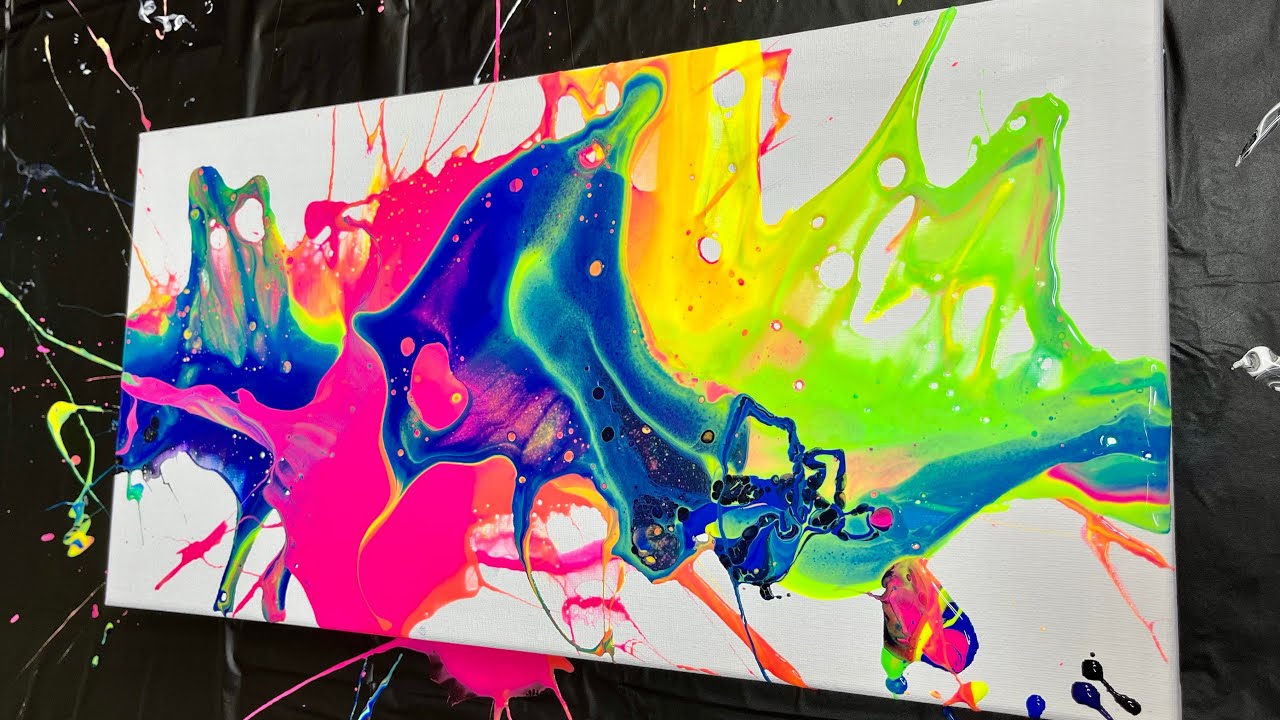This horizontally aligned rectangular painting showcases an abstract, vibrant splatter of colors on a white canvas, reminiscent of an acrylic pour style of art. The painting, also referred to as "painting with a splash," prominently features amorphous, fluorescent splashes and streaks of various colors. In the lower left corner, there is a vivid pink splash, transitioning upward to blue in the middle and yellow above it. The right side exhibits green splatters, with a prominent yellow-green area in the upper right corner. The colors meld together, creating a swirling effect, occasionally evoking the appearance of an astronomical image.

The canvas is mounted on a background that is solid black on the left side, transitioning to a dark gray, rock-like texture on the right. Paint splatters extend beyond the confines of the canvas, creating a dynamic sense of movement. Notably, a tiny bird head appears to emerge from the middle of the right side, pointing its beak towards the artwork. Additionally, the splatters and droplets extend to a black tarp beneath the canvas, indicating the energetic process of its creation, further emphasized by a large pink blob at the bottom. This mesmerizing piece of fluid art, created with squeeze bottles, embodies a vivid, freeform expression without discernible shapes or symbols, making it a captivating sight.